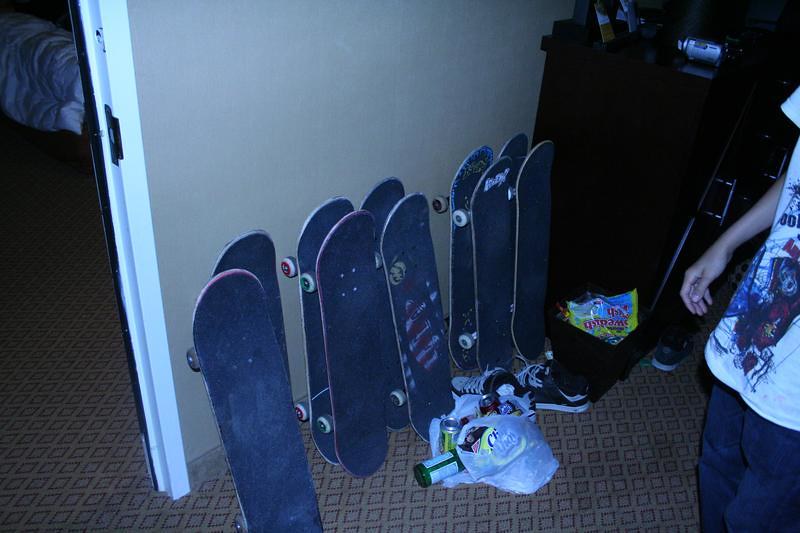Inside a dimly lit room with a gray wall and a dark brown carpet with a diagonal diamond pattern, there are ten skateboards leaning up against the wall in two neat rows of five. The skateboards are primarily navy blue with white wheels, and some have green or red trim. In front of the back row of skateboards, a white plastic bag lies on the floor, containing a green glass bottle and a couple of cans, one of which is yellow. Also scattered in front are a pair of black tennis shoes and a small candy bag. On the right edge of the image, there's a partial view of a person wearing dark blue pants and a white short-sleeved t-shirt with a red and blue graphic. Their right arm is slightly outstretched. To the left, a white doorway frame leads to another room, though its interior is not visible.